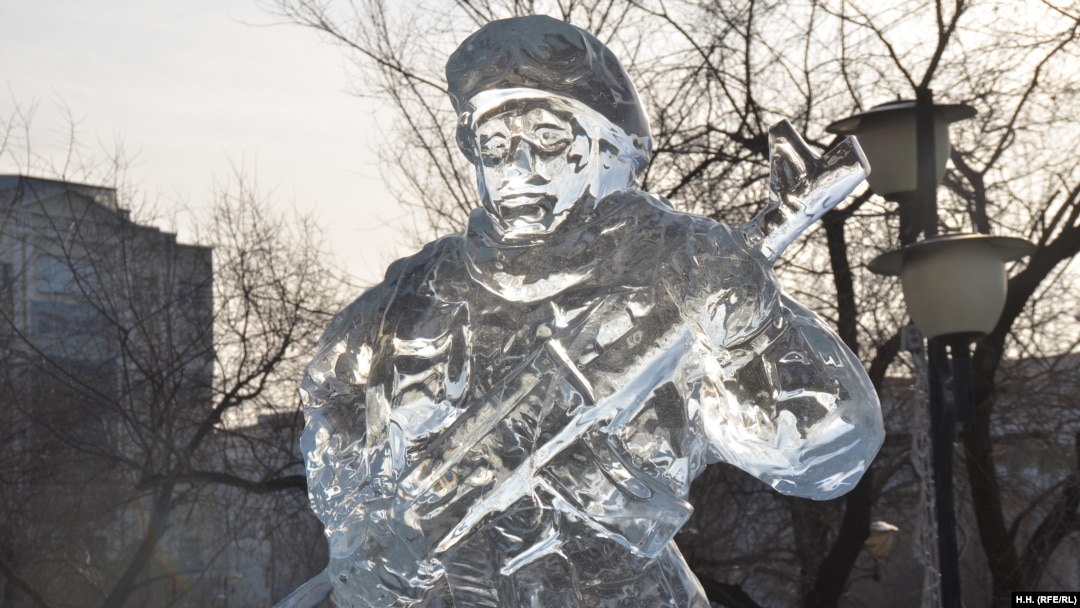The image, taken in muted colors and wintry light, captures an outdoor scene with a towering ice sculpture as the central focus. The landscape-oriented photo shows a city park or similar setting, with bare trees and two lampposts visible in the background. The sculpture, larger than life, depicts a soldier with a helmet and goggles, giving an impression of military attire. The figure, made of clear, translucent ice, is holding an object that could either be a weapon or a guitar, with details like an ammunition sash crossed over the right shoulder enhancing its soldierly appearance. Surrounding the sculpture are grayish light conditions, suggesting a late autumn or early winter time frame, just before dusk. There’s an outline of a building on the left, adding depth to the composition. The bottom right of the image features an unreadable signature. Overall, the photo evokes a cold atmosphere, hinting at a location in a very chilly part of the world, possibly Russia or Siberia.